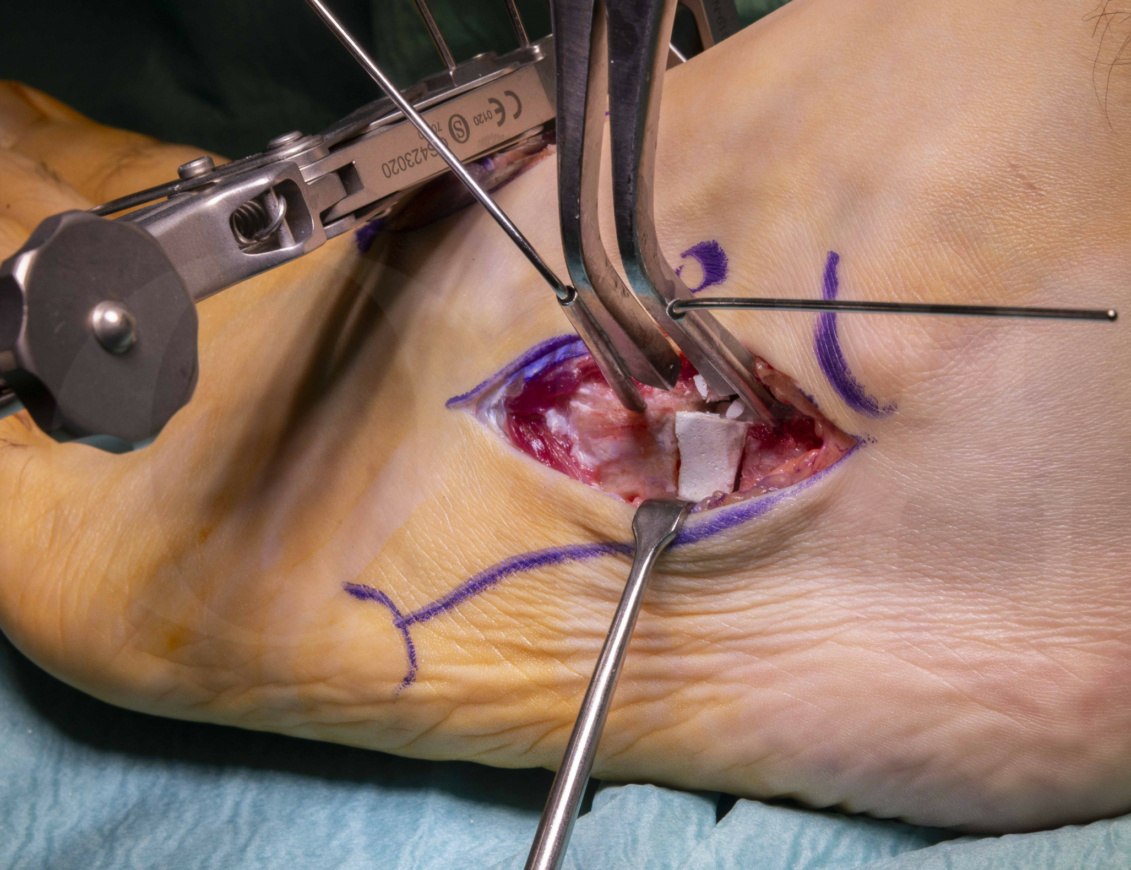This image is a close-up of a surgical procedure on someone's limb, possibly a foot or thigh, as context is limited. The focal point is an elongated, leaf-shaped incision marked with a purple marker on fair skin. The incision area reveals pinkish muscle tissue, white structures that may be bone or surgical material, and is surrounded by blood.

Multiple silver instruments are at work: one thin, rod-like tool is holding the skin open from the top, while another similar tool supports the bottom. Additionally, a wider tool with a numbered dial can be seen at the top of the image, further assisting in the procedure. The area around the incision shows signs of advanced age, indicated by sagging skin and fat. In the upper right corner, a glimpse of brown hair suggests this might be a man's limb. The background features a light blue drape, and the operation appears to be taking place under meticulous care with precision instruments.